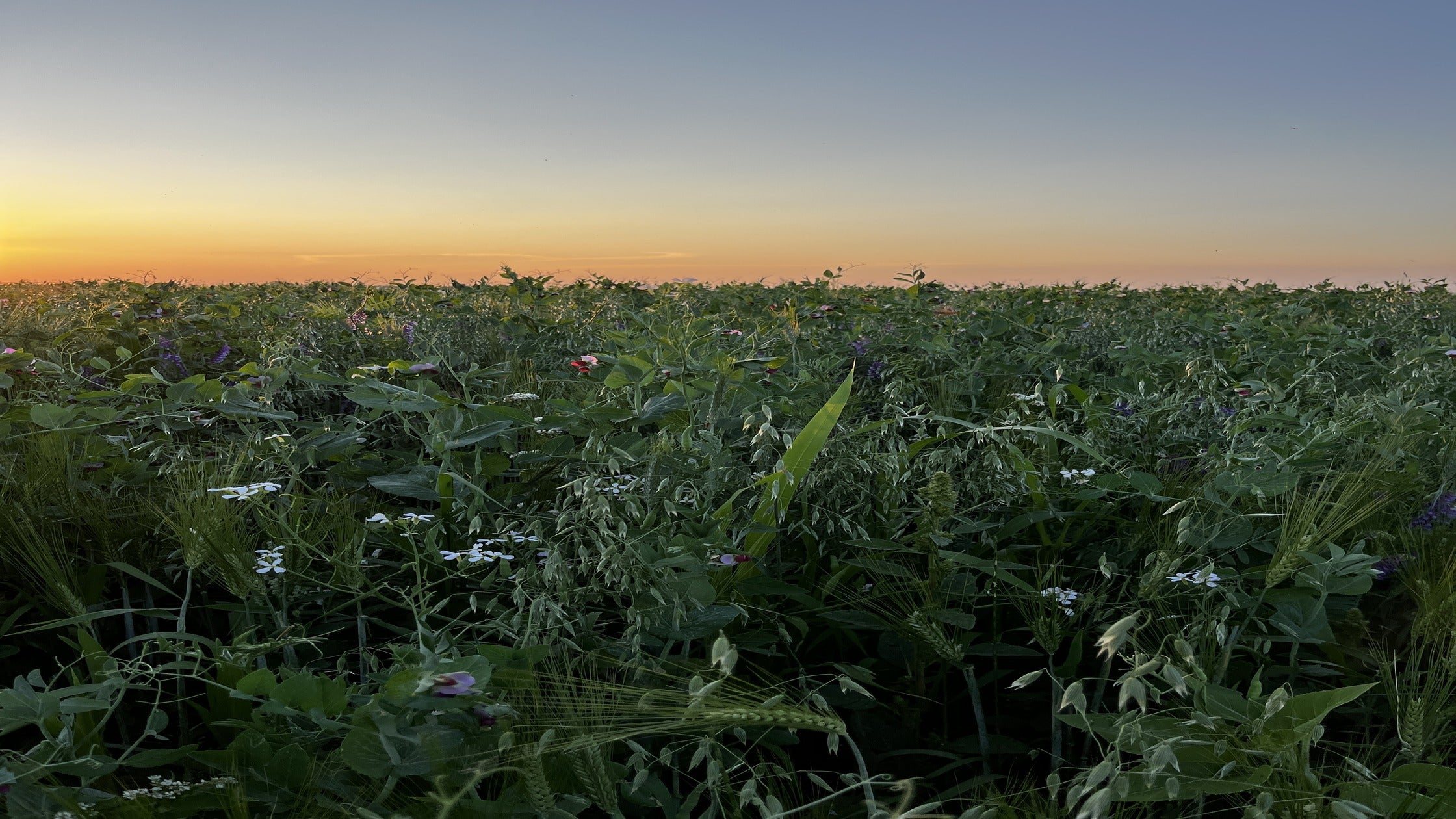The image is a full-color, horizontally rectangular landscape photograph taken outdoors during either sunrise or sunset, utilizing natural light. The top third of the image features a sky that transitions from a soft blue at the very top to a warm orangish-yellow closer to the horizon, hinting at the sun's glow from the far left. The horizon line reveals a sprawling, lush field stretching across the frame, dominated by a verdant tapestry of various green grasses and plants. The field appears untamed, with no discernible rows or organization, suggesting it might be an expanse of wildflowers and grasses rather than an orderly crop. Among the greenery, small clusters of white flowers with four petals are scattered throughout, and a few purple and possibly reddish-pink wildflowers add splashes of color closer to the left and the background. The photo's overall impression is one of serene natural beauty, capturing the tranquil moment of dawn or dusk over a wild and diverse field.